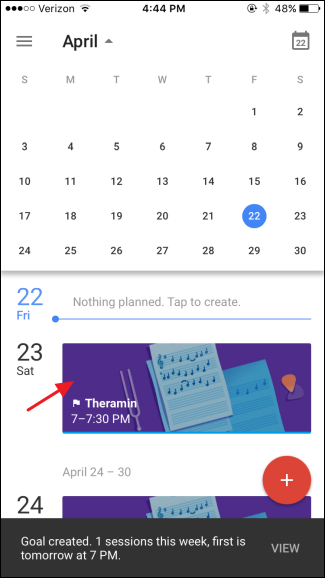The screenshot showcases the Google Calendar app interface on a smartphone. In the top-left corner, it displays the signal strength with three out of five service bars, represented by three filled black dots and two unfilled black outlines. Adjacent to this, "Verizon" is indicated, followed by a Wi-Fi symbol showing moderate to strong connectivity. The current time is displayed prominently in the center as "4:44 PM."

To the left beneath the time, there are three horizontal gray lines symbolizing a dropdown menu. Next to it, the month "April" is printed in bold black text. Further right, a gray arrowhead points upward, followed by a gray calendar icon featuring the number 22. Below it, days of the week abbreviated as SMTWTFS (Sunday through Saturday) are listed in light gray. Starting from Friday (F), the calendar dates range from the 1st to the 30th, with the 22nd prominently highlighted inside a blue circle, indicating the current date.

At the bottom of the screenshot, a shadowy divider can be seen. Towards the top-left under the divider, the number "22" is presented with "FRI" in blue underneath, denoting the day and date. A thin line with a blue dot at the end stretches across the screen. Above this line in gray text, it says "Nothing planned, tap to create." Below, "23 SAT" is written in black font and an arrow points towards a dark purple banner featuring musical notes and a white flag in its bottom corner. The banner text reads "THERAMIN, 7 to 7:30 PM," indicating a scheduled event.